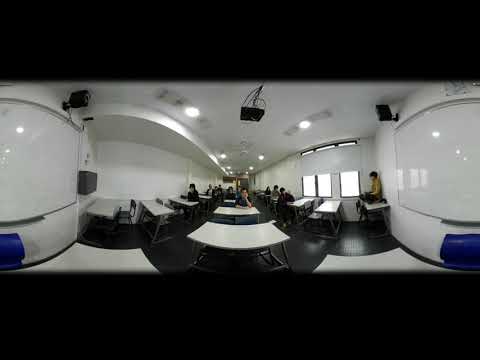The image depicts a semi-empty cafeteria or waiting area, characterized by its white walls and tables, coupled with a contrasting black floor. On either side of the space, two dry erase boards are mounted, accompanied by blue receptacles below them. The ceiling is adorned with lighting fixtures and speakers that emit light beams. In the background, people are seated at various metal-framed white tables, while to the right, a person is seen sitting cross-legged atop a table. The scene appears slightly distorted, as if viewed through a fisheye lens, emphasizing the room’s perspective. This spacious area, possibly a classroom, meeting, or training space, facilitates congregation and work activities, reflecting a clean and modern environment.